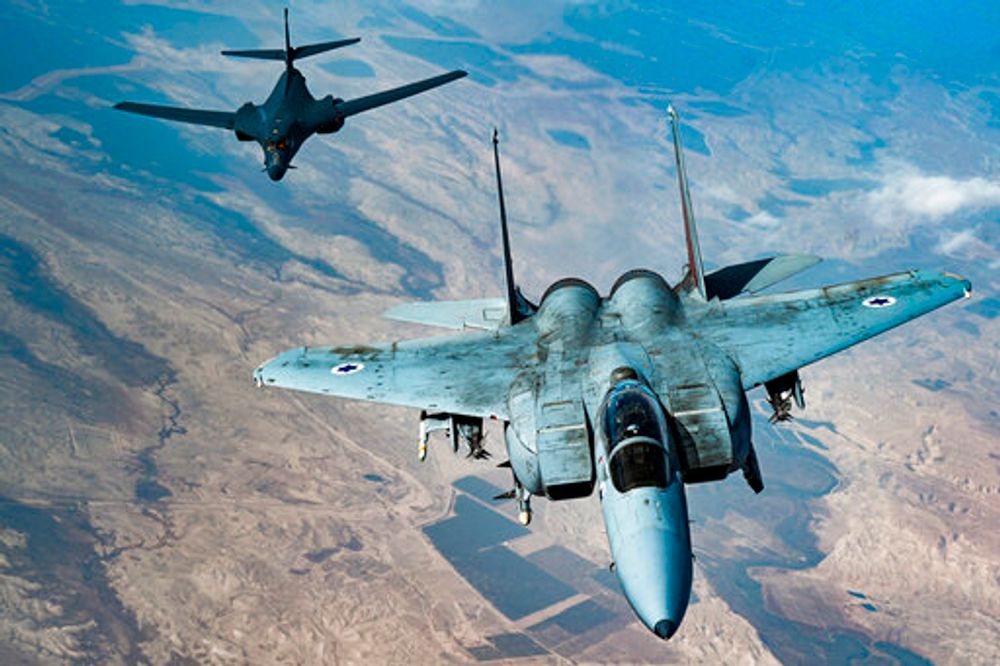In this top-view aerial photograph, we see two military aircraft flying over a remote, valley landscape characterized by beige and dark gray hues. The image, captured in a landscape layout, features a distinct V1 military aircraft towards the center. To the upper left of the image is a darker, almost black jet with a stubby nose, which seems to be trailing behind slightly. In contrast, the lower right showcases a gray-colored fighter jet, with a glass dome revealing a seated pilot inside. Both jets are flying in the same direction, with their noses pointed toward the front of the image and their tails toward the top. The background reveals a desolate, uninhabited valley visible beneath them, and the right side of the image has some cloud coverage, adding to the overall atmospheric detail. The distinct visual distinction between the two jets highlights the military setting of the photograph.